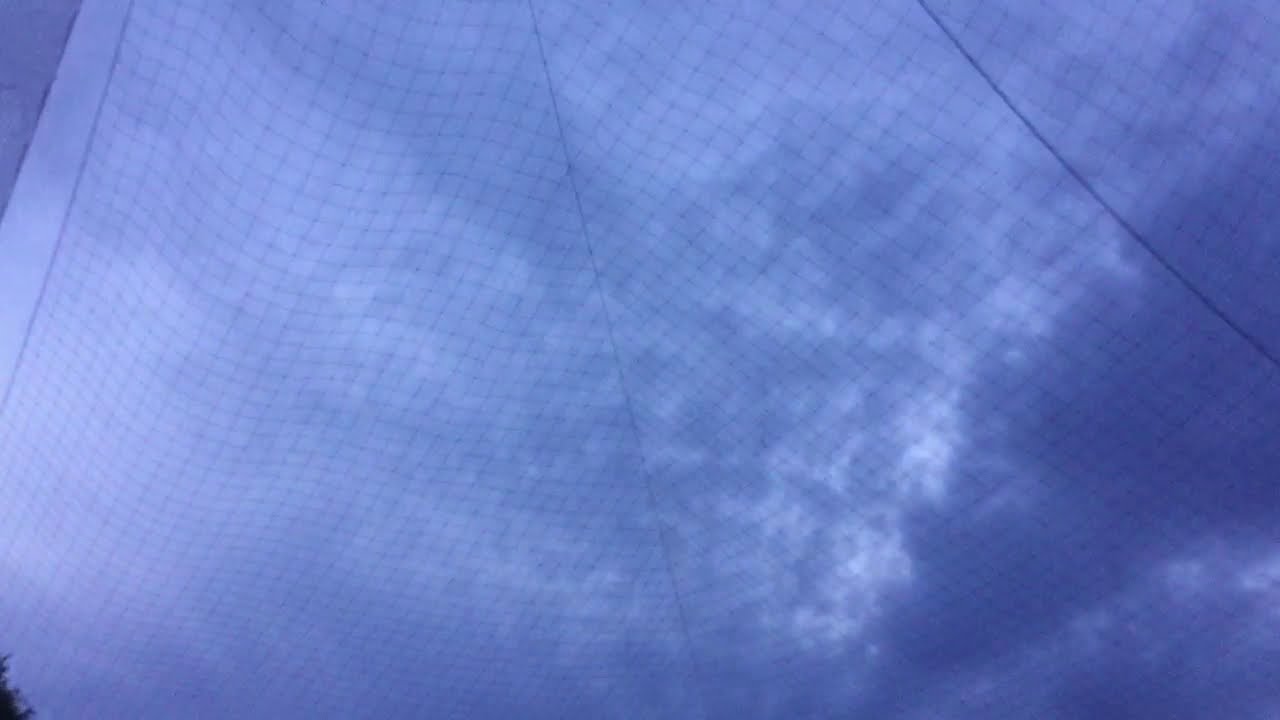The image captures a scene of an overcast sky, framed through a black, grid-style nylon net that covers the entire shot. Through the netting, which is prominently displayed with thicker and thinner segments, the sky is visible, featuring a variety of cloud formations. These clouds, mostly gray with a blue tone, scatter across the sky and create a hazy, almost smoky appearance. The right side of the sky is filled with thicker, darker clouds forming a dense cluster, while the left side exhibits lighter clouds and a less intense blue hue. Dominating the background, this cloudy sky is set against the backdrop of the net, giving the impression that the photo was taken from beneath it.

In the bottom left corner of the image, part of a tree is barely visible, adding a natural element to the composition. The entire scene feels both muted and textured, with the net’s intersecting lines creating a pattern of squares over the cloudy expanse. The image is rectangular, almost twice as wide as it is tall, adding to the expansive feel of the sky. The net's seams are visible, with one seam angling from the top left towards the right bottom, and another forming a triangle with the upper right corner. These seams contribute to the overall grid pattern that characterizes this outdoor snapshot.